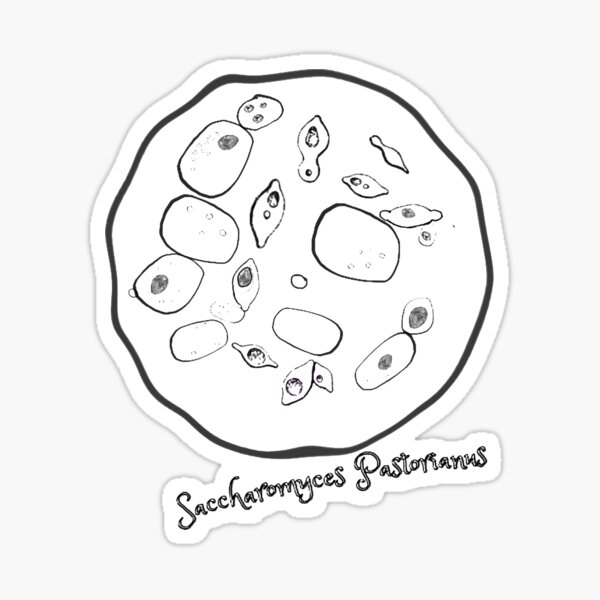This image appears to be a hand-drawn, black-and-white vector illustration resembling a micro-organism or cell, specifically Saccharomyces pastorianus, and it has been made into a sticker. The central circular design features irregular, wavy black outlines filled with various shapes such as squares, oblongs, and pill-like forms, indicative of cellular structures like food vacuoles, mitochondria, and potentially a nucleus, all emphasized by black centers or outlines. The sticker maintains a white border that shapes around the cell's design, enhancing its sticker-like appearance. Underneath this cellular illustration, the name "Saccharomyces pastorianus" is prominently written in black on a white background. The image appears to be placed on a grey or white table surface, suggesting it might be for sale or display.